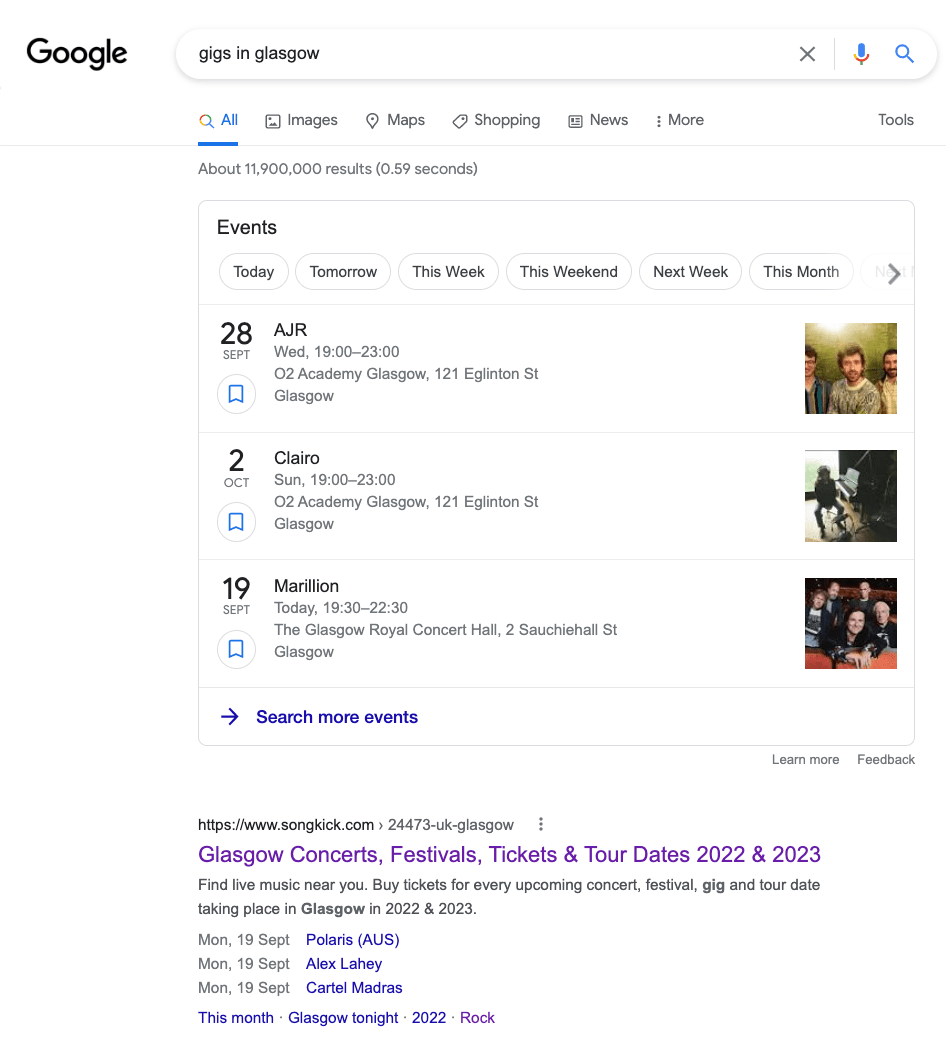This image is a screenshot of a Google search page with a white background. At the top left corner, the "Google" logo is displayed in black. Below the logo, there is a search bar containing the query "gigs in Glasgow." Underneath the search bar are various tabs: "All," "Images," "Maps," "Shopping," "News," and "More," with the "All" tab currently selected. 

The search results begin with an "Events" section, providing buttons to filter results by different time frames: "Today," "Tomorrow," "This week," "This weekend," "Next week," and "This month." 

The first event listed is on 28 September, featuring AJR, scheduled for Wednesday from 19:00 to 23:00 at the O2 Academy Glasgow, located at 121 Eglinton Street. This entry includes a photograph of the band.

The second event is on 2 October, featuring Claro, scheduled for Sunday from 19:00 to 23:00 at the O2 Academy Glasgow, the same address as above. This entry includes an image of the artist.

The third event is on 19 September, featuring an artist whose name appears to be "Marion" or "Marilyn" (text is unclear). This event takes place today from 19:30 to 22:30 at the Glasgow Royal Concert Hall, accompanied by an image of the band.

Beneath these listings, there is a blue link that says "search more events."

Further down, there's a link to a page titled "Glasgow concert festivals tickets and tour dates 2022 and 2023." This section promotes finding live music near you and buying tickets for upcoming concerts, festivals, gigs (with "gig" in bold), and tour dates.